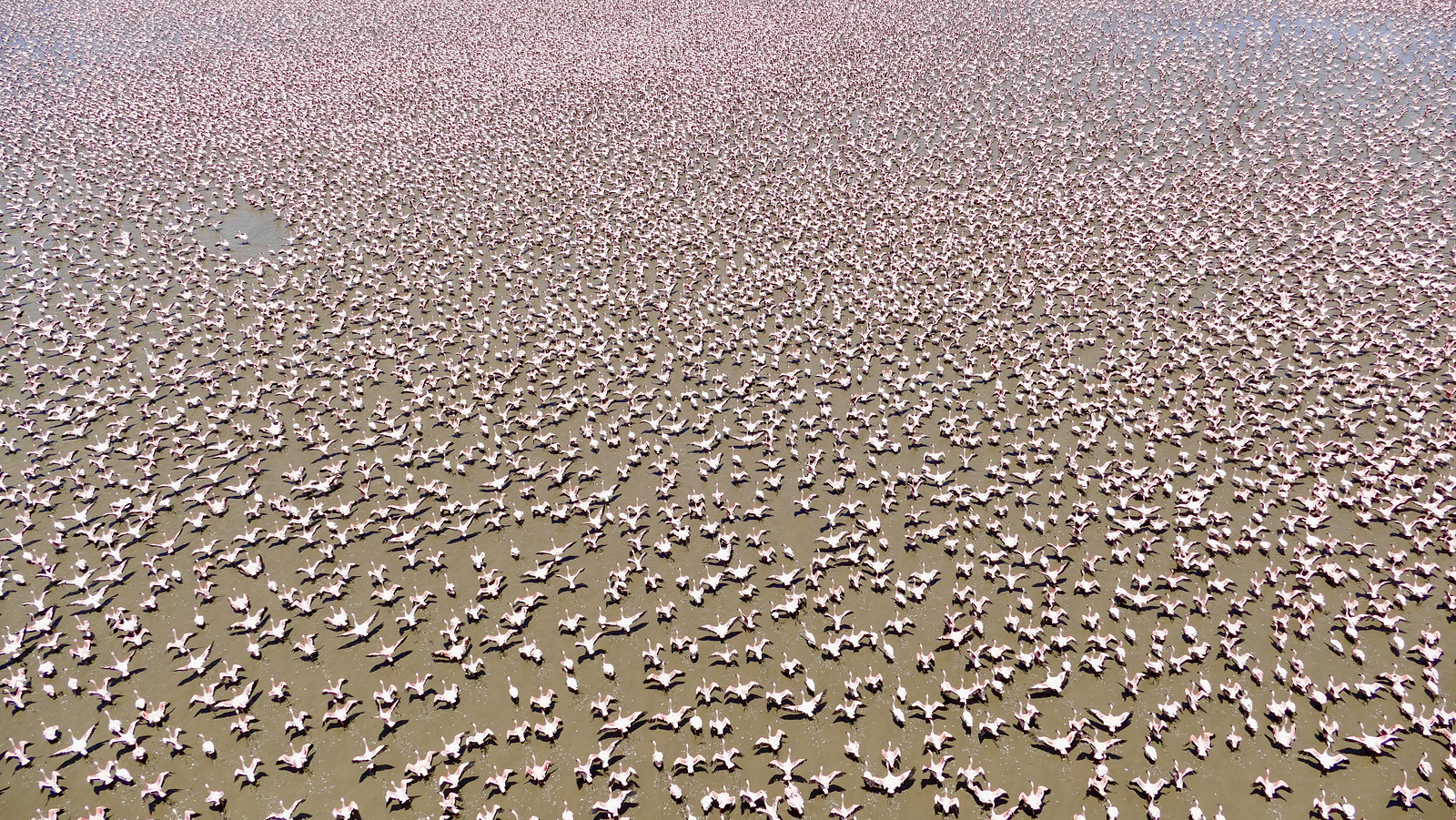This aerial photograph captures a vast assembly of flamingos, possibly thousands, standing close together in shallow, muddy brown water. The image, likely taken from a helicopter or airplane at a slight angle, reveals flamingos appearing larger and more distinct in the lower half, while they condense into a pinkish mass towards the upper portions. The water is uniformly brown except for a reflection of the blue sky in the top right corner. The scene hints at a potential migration, with the birds densely populated except for a sparse area in the top left quadrant. The flamingos, characterized by their white and pink hues, resemble pink specks on a beige background when viewed from a distance, creating a mesmerizing pattern across the expanse. The photograph, taken in daylight, perhaps at noon, bathes the entire scene in a gentle, direct sunlight.